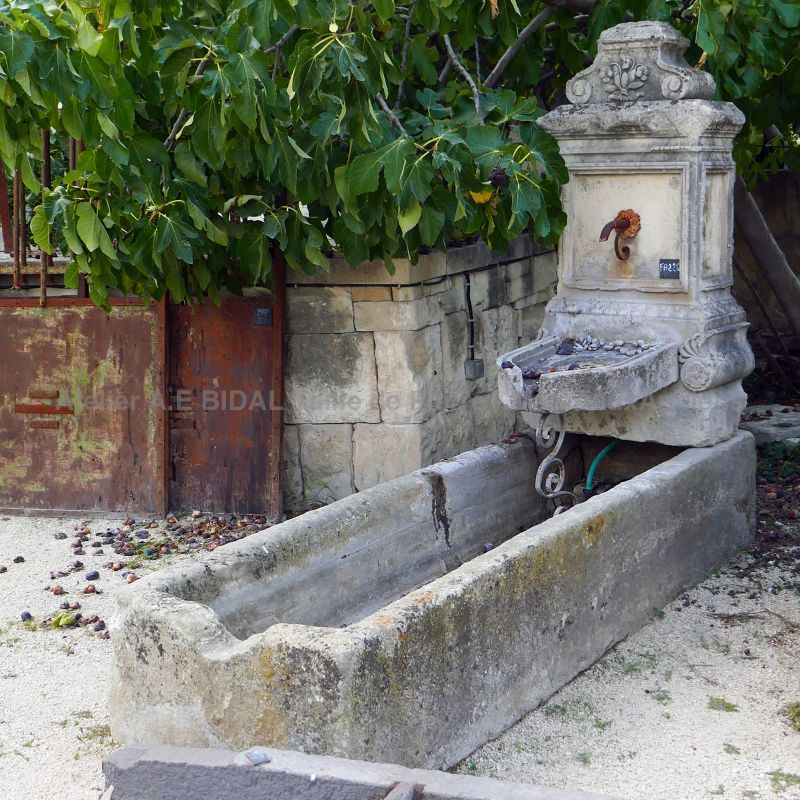The outdoor photograph showcases an aged concrete fountain with a bronze or copper spout located at the right side of the image. This spout elegantly curls and appears slightly rusted. Below it, there's a semi-circular stone basin that fills with water, which then overflows into a larger rectangular trough. The entire fountain structure has noticeable discolorations, particularly green around the edges, and some areas where the concrete has chipped away. 

To the left of the fountain, a brick wall covered in overgrown plants and leaves can be seen. The wall extends to a rusted fence or railing that's mostly obscured by the greenery. Scattered on the rocky ground in front are white pebbles along with fallen nuts and berries from the trees in the background. A green hose is also visible near the base of the fountain. Additionally, a semi-transparent watermark reading "Atlir A.E. Bridal" is present across the center left of the image.